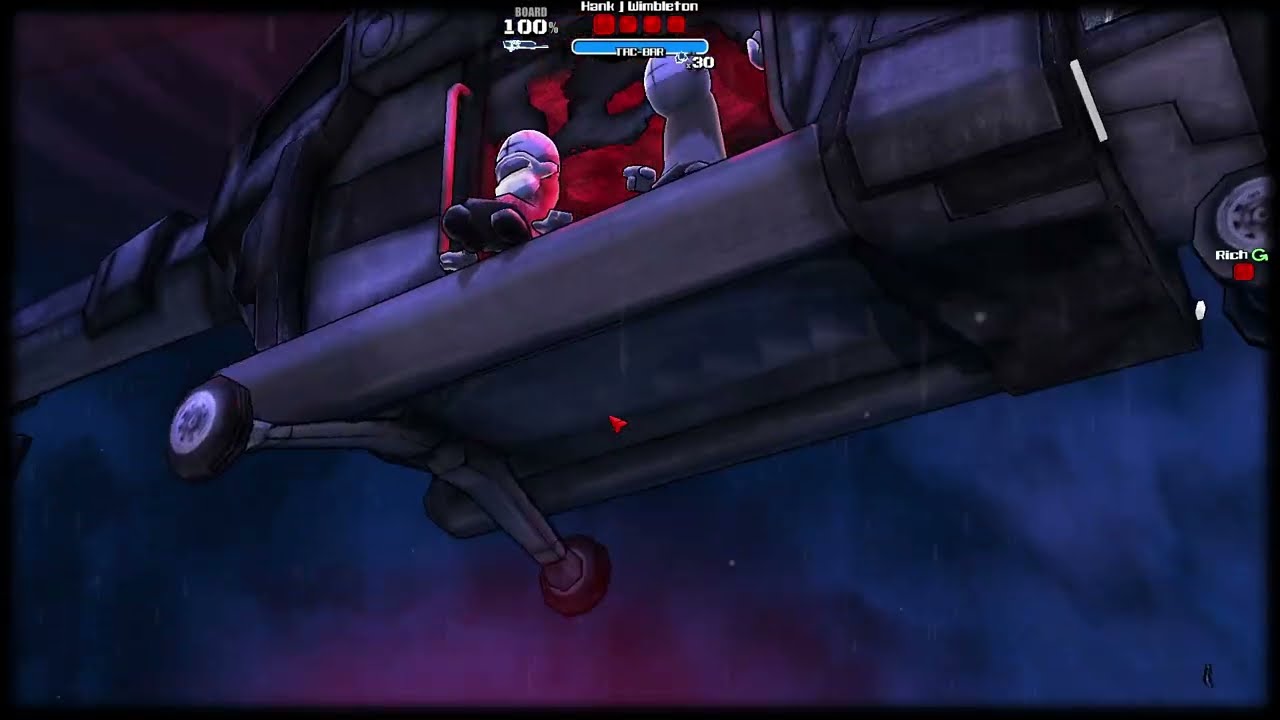The image depicts a nighttime scene from a video game, presented in a stylized, cell-shaded 3D animation. A low angle shot reveals the underside of a helicopter with realistic proportions but a cartoony feel. The sky above is a dark blue with hints of pink and red, suggesting nightfall. The helicopter's side door is open, and it is illuminated by a red interior light. Inside the helicopter are two peculiar figurines. The one on the left appears to have a rounded head with a cross shape and blocky, robotic hands, and seems to be wearing a mask or helmet while sitting with crossed legs. The other figure, similarly outlandish, has a plump, square shape with hands and feet sticking out from beneath what looks like a robe. The screenshot also includes game interface elements: at the top center, there is a health bar along with an ammunition indicator showing '100%'. The name 'Hank J. Wimbleton' is written in white above these stats, and it looks like it could be from a combat or shooter game. Additional details include the presence of rain, visible helicopter wheels, and a curved square shape around the helicopter's tail.